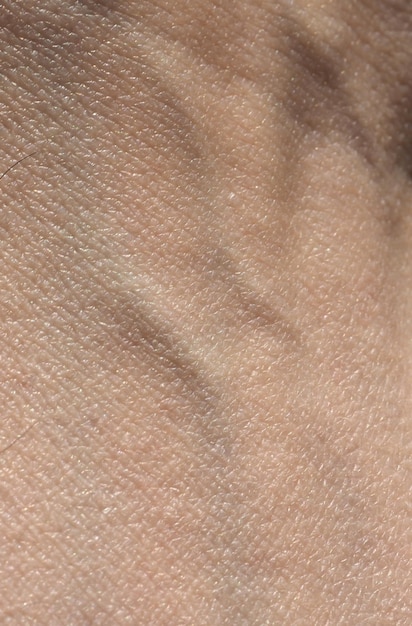This image is an extreme close-up of human skin with a detailed focus on its texture. The skin appears to have a fair to tan-pinkish complexion, capturing the fine striations, pores, and subtle blemishes on the surface. Two fine black hairs are visible on the left side of the image, and the skin texture becomes rougher toward the upper right corner. Central to the photo are two prominent veins, with one vein forming the shape of a soft 'Z' and another resembling a wave. These veins subtly protrude, adding depth to the otherwise smooth surface. The image is enclosed within a vertical rectangle and is illuminated by a light source, though it's unclear whether this is taken outdoors or indoors. The intricate detail highlights the complex and diverse nature of human skin.